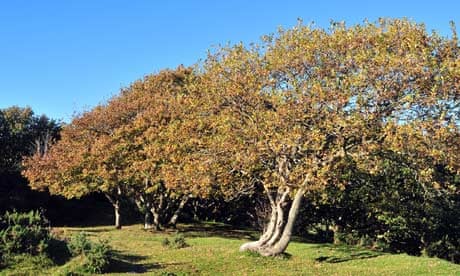In the middle of a sprawling, grassy area that looks well-mowed but thinning in some areas, stands an impressive tree with a fascinating structure of three gnarled and somewhat curvy trunks branching out from a shared, large root protruding from the ground. The massive canopy of leaves above displays a palette of brownish-red, yellow, gold, green, and orange hues, indicative of autumn. To the left of this unique tree is another similar but slightly less distinctive tree, also featuring numerous trunks and expansive, leafy branches. The grassy area is punctuated with patches of overgrown weeds and scattered grass clippings, especially towards the bottom left corner. The backdrop is a bright, vibrant blue sky on a sunny day, framing the scene with a quintessential autumnal vibe. The quality of the image may not be the crispest, but the vivid details and colors of the trees and their surroundings make the scene richly descriptive. In the background, additional trees and bushes contribute to the feeling of a serene natural landscape.